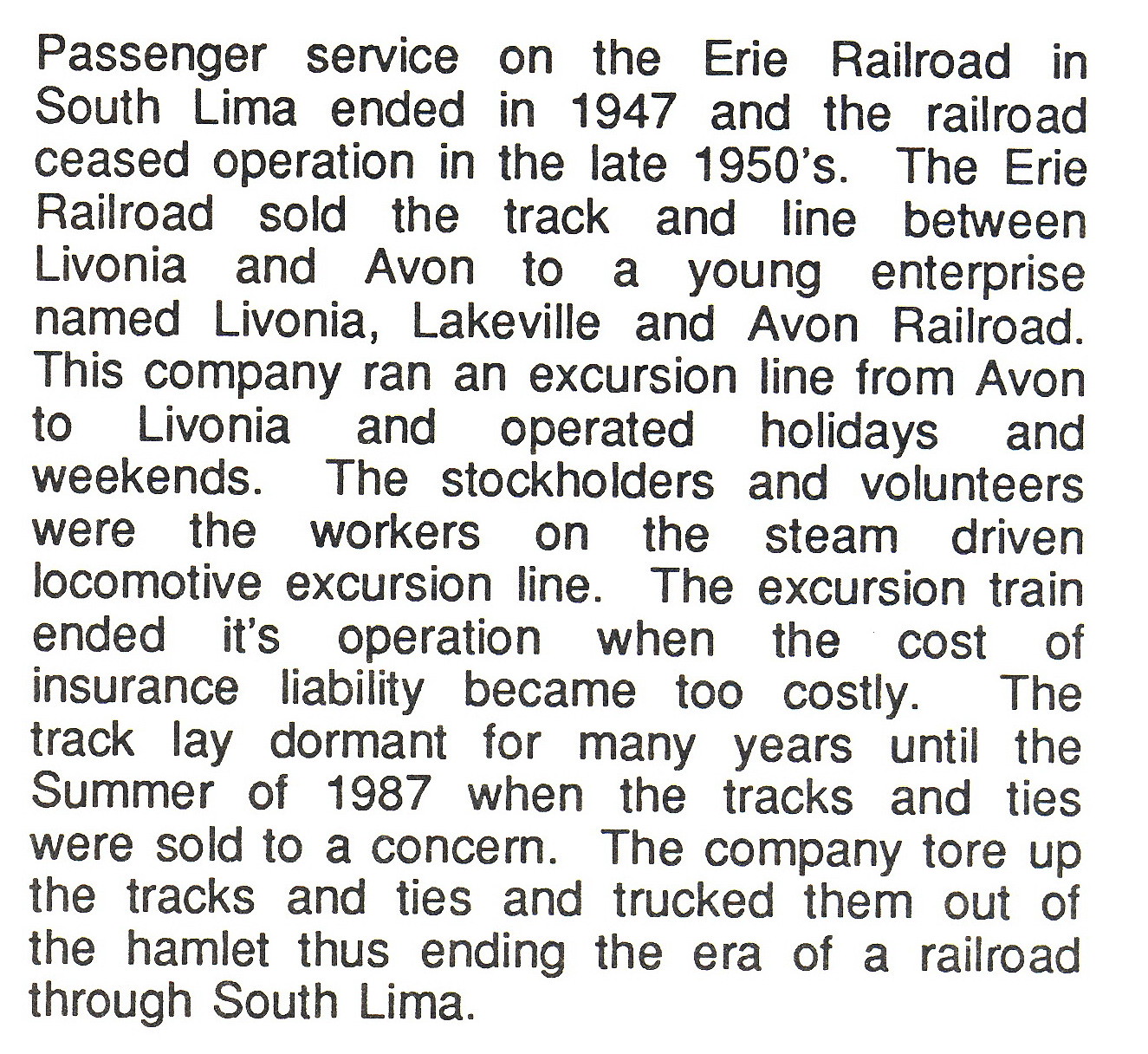The image is a square and features a white background with a large amount of black text, resembling a page from a newspaper. The text details the history of railway operations: Passenger service on the Erie Railroad in South Lima ended in 1947, and the railroad ceased operation in the late 1950s. The Erie Railroad sold the track and line between Livonia and Avon to a young enterprise named Livonia, Lakeville, and Avon Railroad. This company operated a steam-driven excursion train from Avon to Livonia on holidays and weekends, staffed by stockholders and volunteers. The excursion train ceased due to high insurance liability costs. The track remained unused for many years until the summer of 1987 when the tracks and ties were sold to another company, which subsequently dismantled and removed them, marking the end of the railroad era in South Lima.